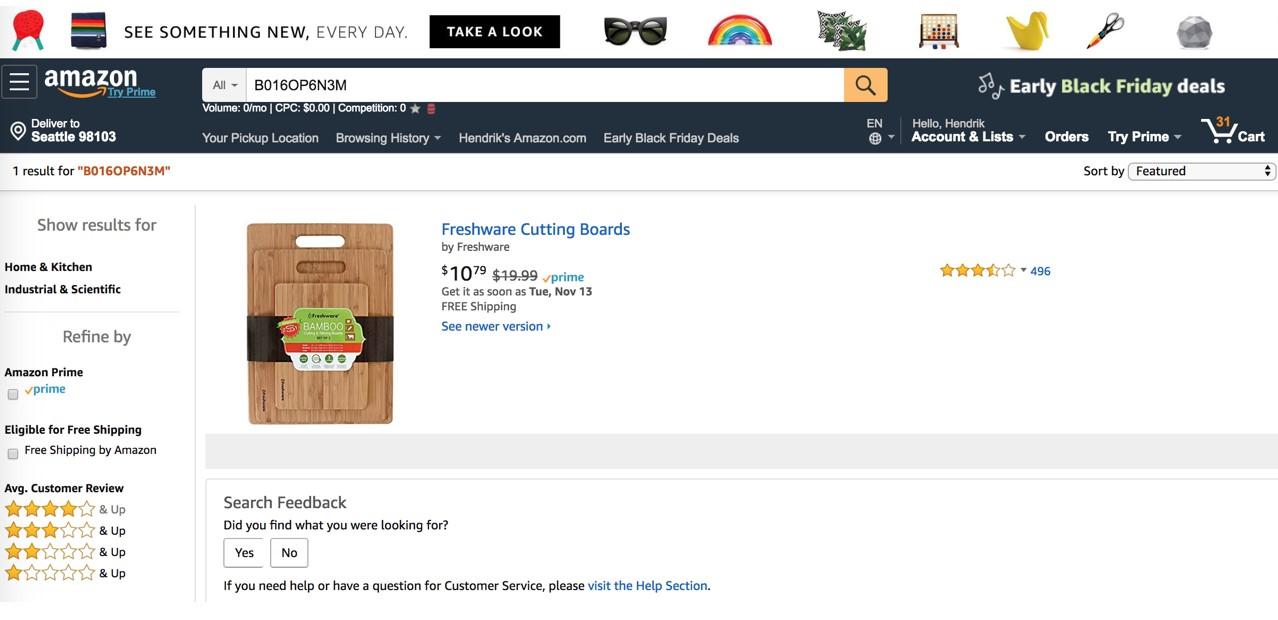This is an Amazon.com product page showcasing Freshware Cutting Boards. The page displays three cutting boards of different sizes: small, medium, and large. The headline reads "Freshware Cutting Boards by Freshware," and the set is priced at $10.79, discounted from the original price of $19.99. Prime members can enjoy free shipping with the promise of delivery by Tuesday, November 13th. A link is provided to view a newer version of the product. To the right, the product rating is displayed, showing 3.5 stars based on 496 customer reviews. 

The left sidebar categorizes the product under "Home and Kitchen" and "Industrial and Scientific," with filtering options for items eligible for Amazon Prime and free shipping. The customer reviews contributing to the average rating are shown, including a 4-star, a 3-star, a 2-star, and a 1-star review, indicating that users can search and sort by these ratings.

The page layout includes the standard Amazon interface with a navigation bar featuring the Amazon logo, a delivery location indicator, a search bar, account and list management options, a shopping cart, and advertisements for early Black Friday deals. Notices such as "Try Prime," "Your Favorite," "Your Pickup Location," and "Browsing History" are also present.